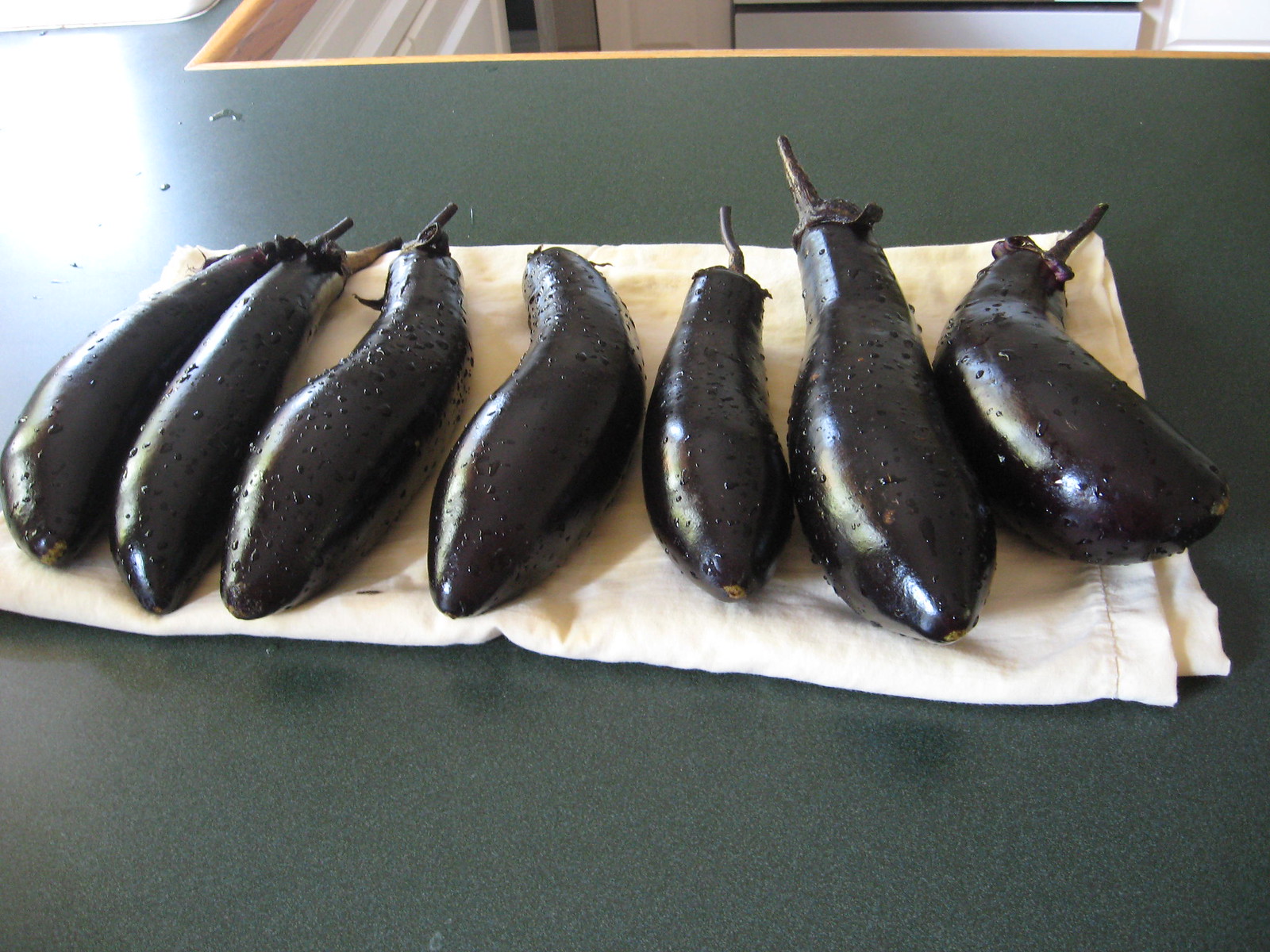The image is taken indoors, showcasing a detailed view of a kitchen counter. The countertop itself is made of greenish-gray Formica with a light brown wood grain trim around the edges. Above the counter, white cabinets are partially visible, contributing to the kitchen setting. 

Prominently displayed on the counter is a thick white kitchen towel, folded lengthwise, stretching from left to right. On top of this towel, there are seven wet, freshly washed eggplants. These eggplants vary in shapes and sizes, with all of them maintaining their stems, which exhibit a slightly lighter purple hue near the attachment. 

The eggplants are characterized by a dark, almost black, glossy surface covered in small black dots, and they glisten under the light due to moisture. One eggplant towards the end is notably curved to the right. Light reflections and water droplets are accentuated on both the eggplants and the countertop, suggesting sunlight streaming into the kitchen. The scene is also marked by shadows cast by the eggplants, adding to the depth and realism of the image.